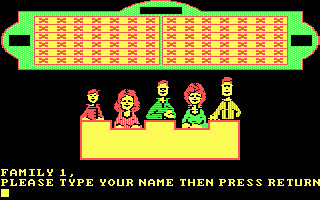This small, rectangular image showcases a screen from the first-generation Family Feud video game, characterized by its pixelated, vintage aesthetic. Dominating the top portion is the iconic Family Feud board, featuring a green background with yellow sections and prominently displaying red X's. Centrally placed is a podium, colored yellow with a red outline, where an animated family stands. The family members, all depicted in yellow hues, are distinguished by varying styles of red hair. A prompt at the bottom reads, "Family 1, please type your name then press return," set against a stark black background. The overall impression evokes a strong sense of early video game design and nostalgia.